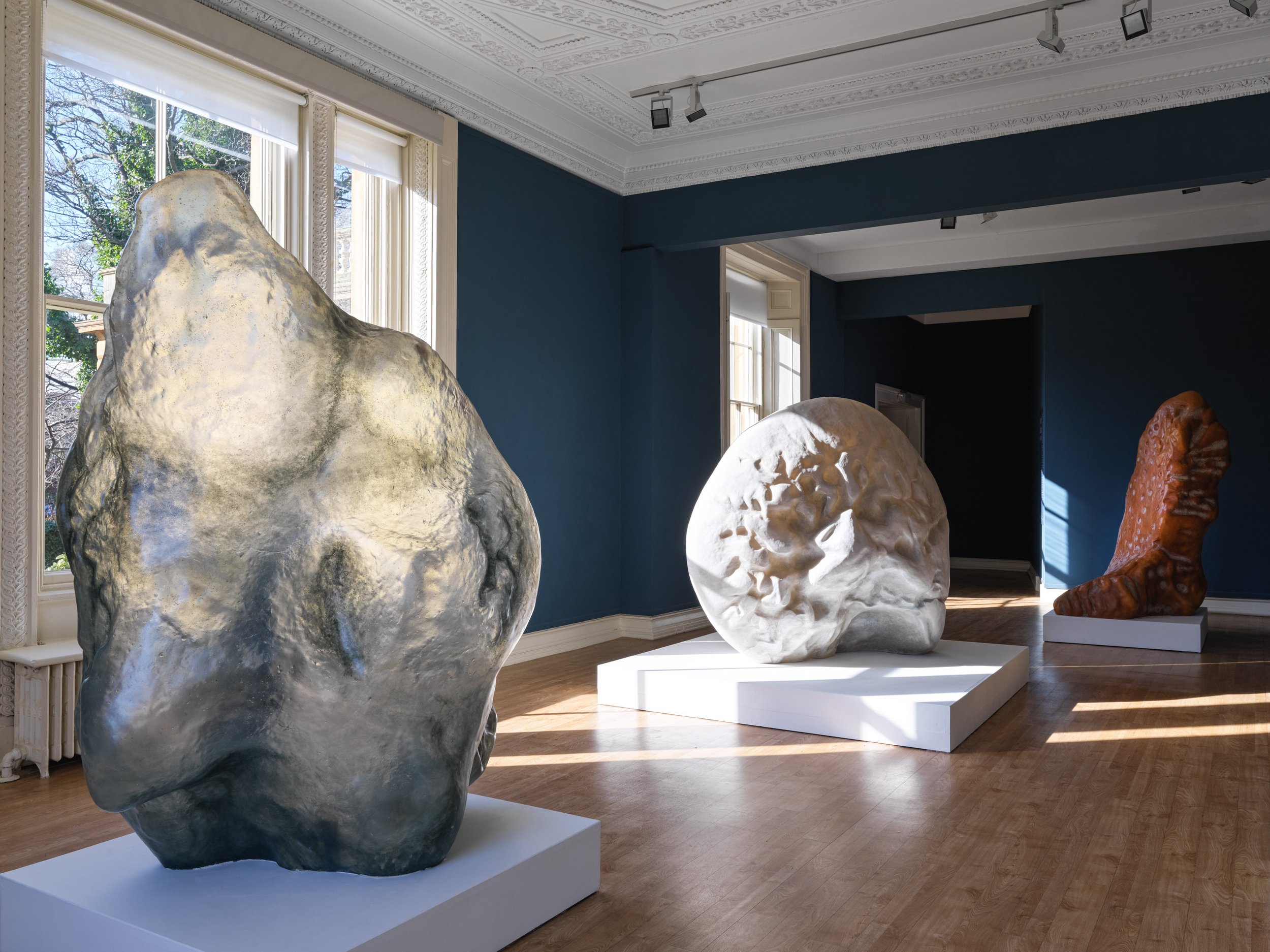This photograph captures an exhibition hall within an ornate, historic museum, possibly dating back to the late 1800s or early 1900s. The room features a richly detailed white ceiling with intricate carvings, complemented by modern skylights that allow additional natural light to filter through. The floor is wooden with a warm, brown hue. Positioned on this wooden floor are several white platforms that display three large rocks, each distinct in shape and color. 

One rock is white and almost spherical, another is red and elongated, while the third is gray-silver with an indefinite, irregular shape. These rocks, potentially made of volcanic material or granite, are presented as art pieces within the museum. The walls of the exhibition hall are a dark blue, with windows that let in daylight, enhancing the dramatic contrast and highlighting the geological displays. The overall atmosphere blends historical architecture with contemporary exhibition design.